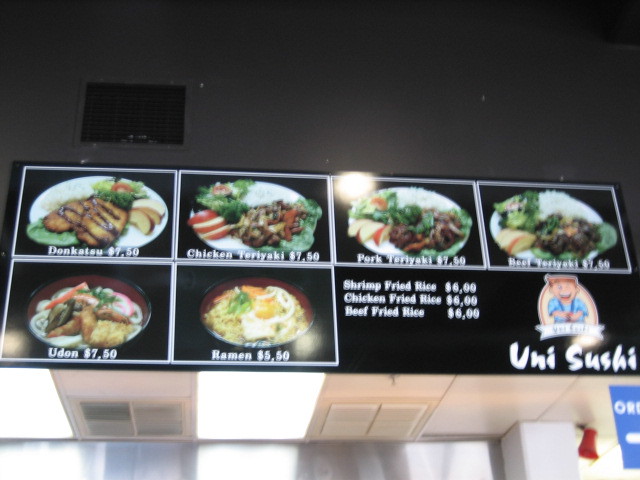The photograph captures a section of a black-painted wall, likely situated above a counter in what appears to be a restaurant setting. The focal point of the wall is a main sign displaying "Uni Sushi," accompanied by an image of a smiling person. Arranged beneath the main sign are six framed photographs, each depicting a different dish offered by the restaurant, complete with descriptions and pricing. The dishes include:

1. Donkatsu - $7.50
2. Chicken Teriyaki - $7.50
3. Pork Teriyaki - $7.50
4. Beef Teriyaki - $7.50
5. Udon - $7.50
6. Ramen - $5.50

Additionally, there are three menu items listed without accompanying images:
1. Shrimp Fried Rice - $6.00
2. Chicken Fried Rice - $6.00
3. Beef Fried Rice - $6.00

Below this wall, a dropped ceiling is visible, featuring vents likely used for heating or cooling purposes, suggesting the photo was taken in a well-maintained restaurant interior. The entire setup provides a clear and inviting overview of the menu specials available at Uni Sushi.